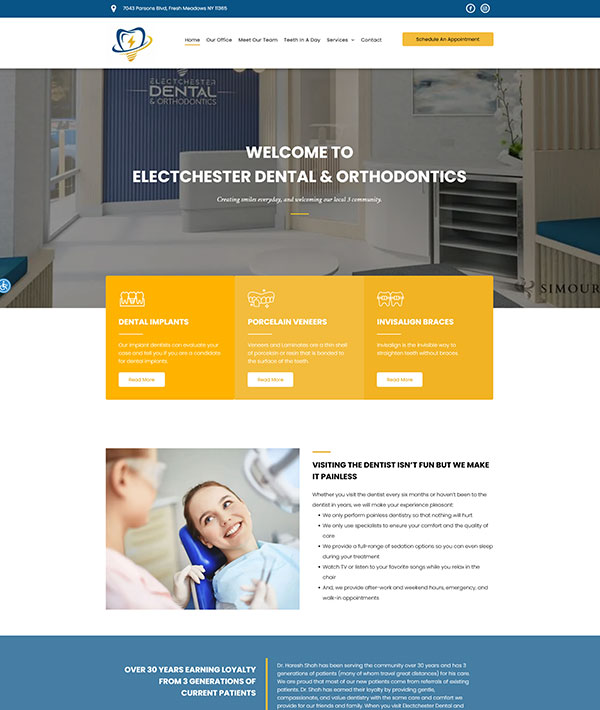The image is a screenshot of the homepage of a dental and orthodontic website for "Alex Chester Dental and Orthodontics." Prominently displayed in the middle of the page is a warm welcome message: "Welcome to Alex Chester Dental and Orthodontics." Below the welcome message, there is a graphic detailing their primary services: "Dental Implants," "Porcelain Veneers," and "Invisalign Braces." Each service is contained within its own box, and at the bottom of each box, there's a white button labeled "Read More." Beneath these boxes, there is an image of a young girl sitting in a dental chair, accompanied by the reassuring text: "Visiting the dentist isn't fun, but we make it painless." Some additional descriptive sentences are present but are too small to read clearly.